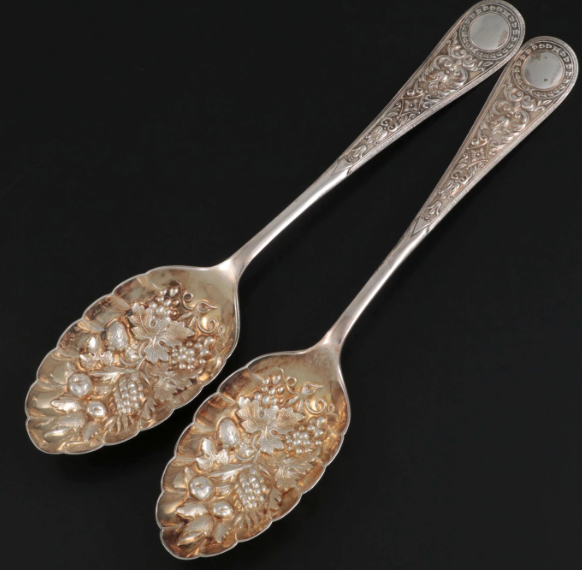On a black background, two ornate silver spoons are displayed. Each spoon features intricate, ornate engravings that extend halfway through the handle up to its end. At the top of the handle, there is a circular area with inscriptions, meticulously surrounded by an engraved ring. The spoon bowls are adorned with shimmering details resembling leaf motifs, grapes, fruits, and other items, enhanced by the unique notches and bubbled edges that give the bowls a cloud-like appearance. The spoons exhibit a bronze-like tarnish, particularly in the areas where they would be used, adding to their antique charm.